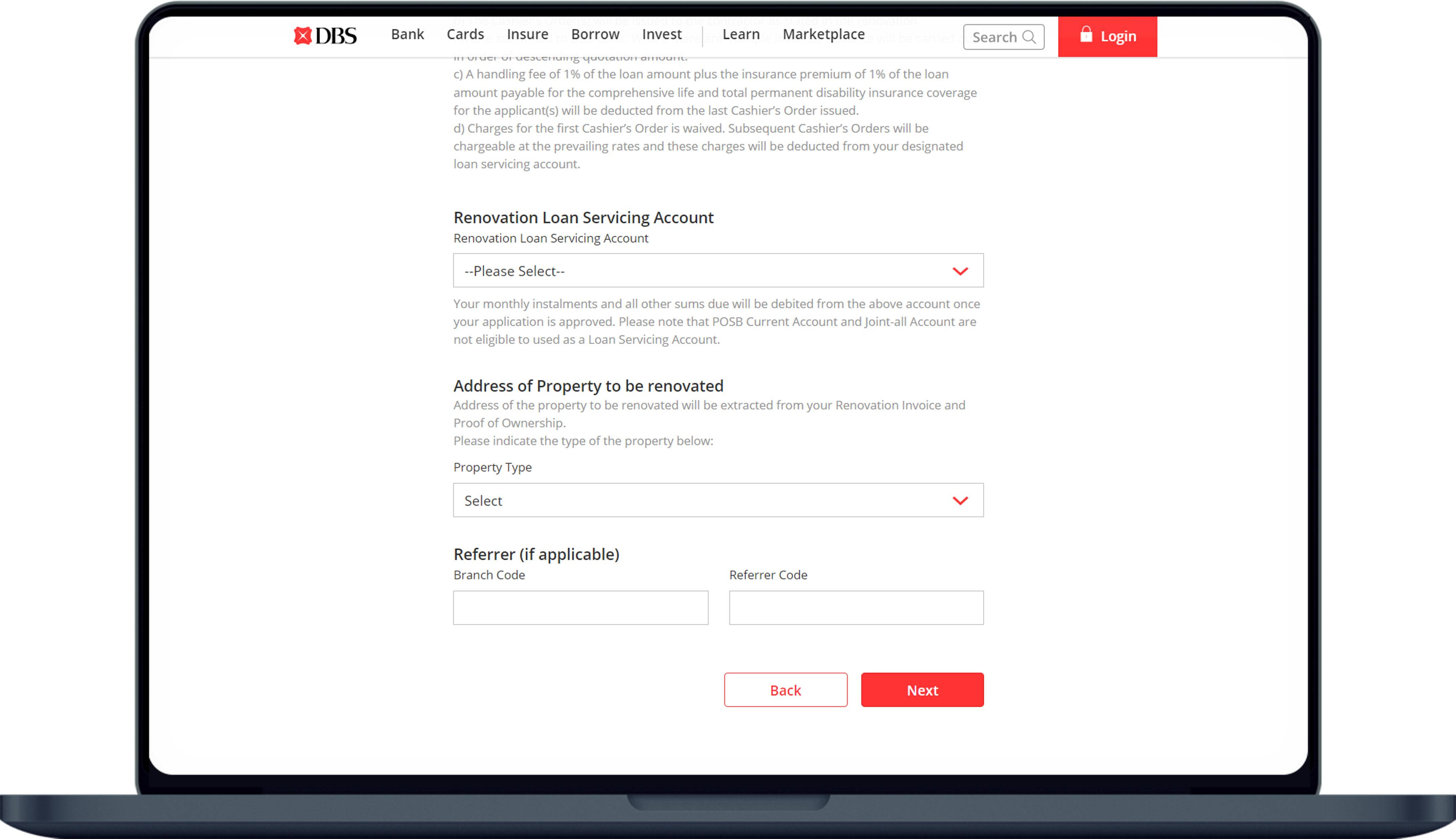An open laptop is displaying a DBS bank webpage. The top navigation bar includes options such as "Cards," "Insure," "Borrow," "Invest," "Learn," and "Marketplace." Below the navigation bar, there is a rectangular search box featuring a magnifying glass icon. Beside it, an orange rectangle button with "Login" written in white text is accompanied by a white lock icon.

The main content area contains information about a "Renovation Loan Servicing Account." It prompts users to input details like the address of the property to be renovated, which will be extracted from the renovation invoice and proof of ownership. The form instructs users to indicate the type of property. There is a drop-down menu labeled "Property Type" and a section for "Refer, if applicable (Branch Code)," with a corresponding input box.

At the bottom of this section, there are buttons for navigation: a gray "Back" button and an orange "Next" button for proceeding to the next step.